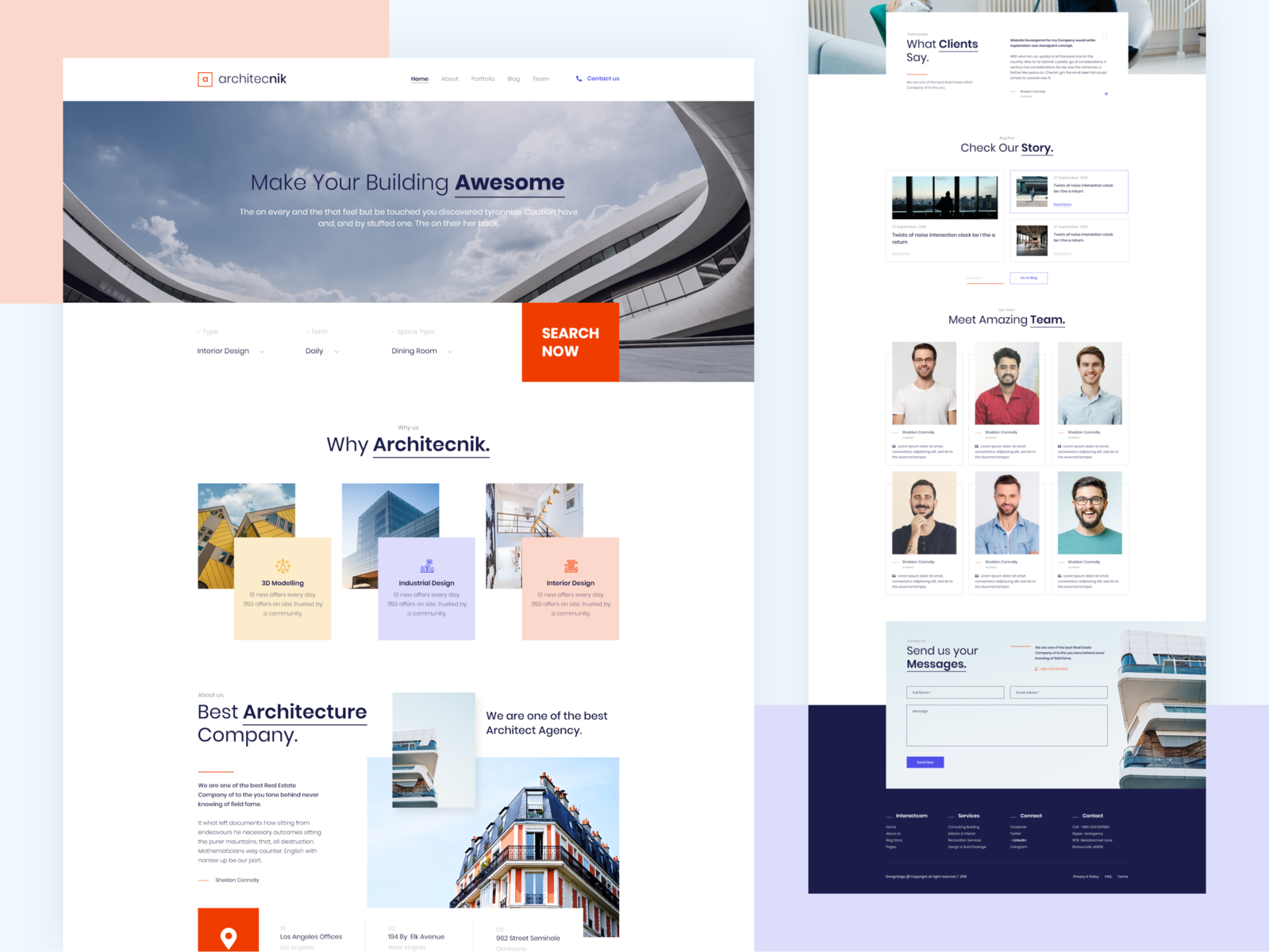The image features a dynamic background with geometric shapes in various pastel colors: a light pink rectangle in the top left, a light blue square covering the majority of the background, and a pale light purple rectangle in the bottom right. 

On the left side, a mock-up of a white web page captures attention. At the top left of the page, the text reads "Architect Nick," accompanied by a logo consisting of an orange "A" enveloped by orange lines forming a square. Below, the navigation menu displays options labeled "Home," "About," "Purchase," "Blog," "Team," and "Contact Us."

The center of the webpage showcases a stunning image of the sky intertwined with a modern building. Beneath this image, a white rectangle contains headings like "Interior Design," "Daily," and "Dining Room," next to an orange button labeled "Search Now."

Midway down the page, bold text asks "Why Architect Nick?" followed by three informational bullet points in separate squares: "3D Modeling" in yellow, "Industrial Design" in purple, and "Interior Design" in peach. Below, a block of text declares, "Best Architecture Company. We are one of the best architecture companies," along with an image of a building and an orange square positioned at the bottom left.

On the right side of the image, a portrait-oriented smartphone showcases client testimonials under "What Clients Say." Further down, the section "Meet Amazing Team" is set against a white background, displaying six portrait thumbnails of the team members of Architect Nick. The bottom of the webpage invites interaction with a form titled "Send Us Your Messages," providing fields for users to fill out their email addresses.